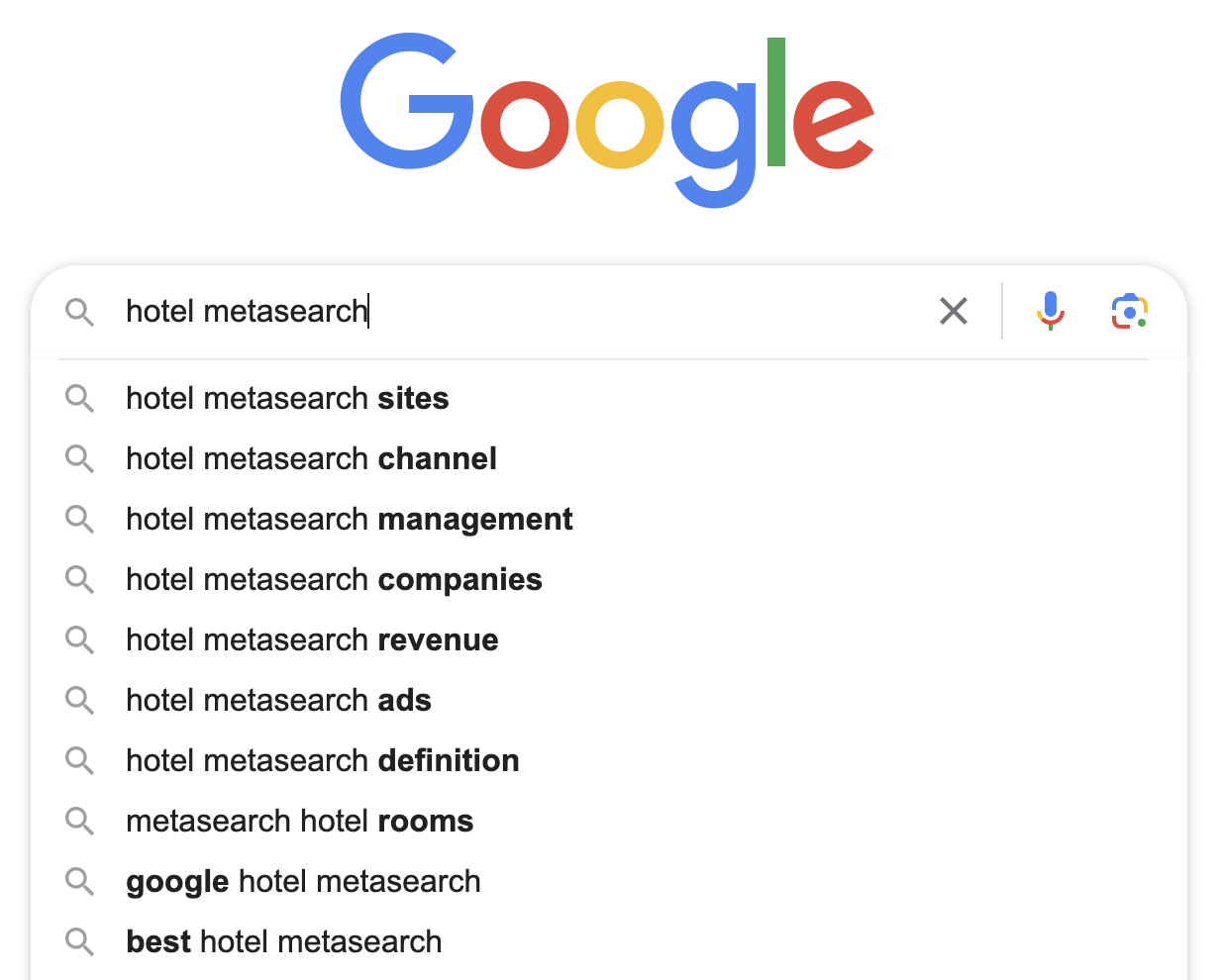The image depicts a Google search page with a classic white background. At the top of the page, the colorful Google logo is prominently displayed. Below the logo is the Google search box with the words "hotel meta search" typed inside. To the right of the search box, there are several interactive icons: a search icon, a microphone icon for voice search, and an icon resembling a camera, which is likely for image search. Further to the right, there's a small 'X' icon used for clearing the search query.

Below the search box, the page lists search suggestions in vertical order, each preceded by a small magnifying glass icon. The suggestions read:
1. hotel meta search sites
2. hotel meta search channel
3. hotel meta search management
4. hotel meta search companies
5. hotel meta search revenue
6. hotel meta search ads
7. hotel meta search definition
8. hotel meta search rooms
9. Google hotel meta search
10. best hotel meta search

The bolded words within these suggestions are "sites, channel, management, companies, revenue, ads, definition, rooms, Google, best," standing out in the search results, indicating their relevance to the query "hotel meta search."